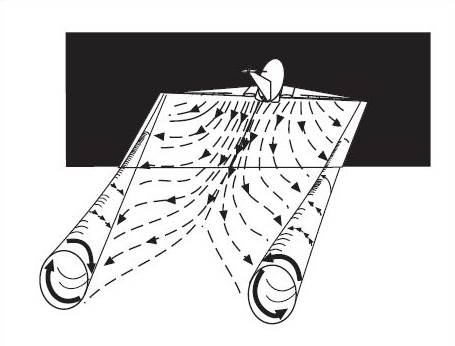The illustration is a detailed black-and-white drawing with a distinct dual-colored design. The top half of the image features a large black rectangle, and at its center, there's an intricate rolled-up paper graphic. This paper appears to encase an egg-like figure with an eye, and from the bottom of the egg, an arm emerges.

From the central rolled-up paper, numerous sketched lines flow downward, adorned with arrow tips. The arrows, starting dense at the top, point downwards but spread out sparser as they travel across the paper's surface. These directional lines create a sense of dynamic movement, as if illustrating a force or flow.

On both ends of the paper, depicted like circular tubes, there are arrows indicating rotational motion: the left tube's arrows move clockwise, while the right tube's arrows move counterclockwise. Separately, an additional black arrow is drawn moving to the right from the top of the left tube.

The entire design may convey the concept of wind movement or drag over an object, possibly an airplane, suggested by the contours and flow of the arrows that reflect a vortex-like pattern. At the top of the illustration, where the black and white sections converge, a small satellite dish-like element is visible, potentially symbolizing the origin point from which all the lines and arrows emanate. This compelling artwork merges technical and abstract elements to depict a dynamic flow of forces.